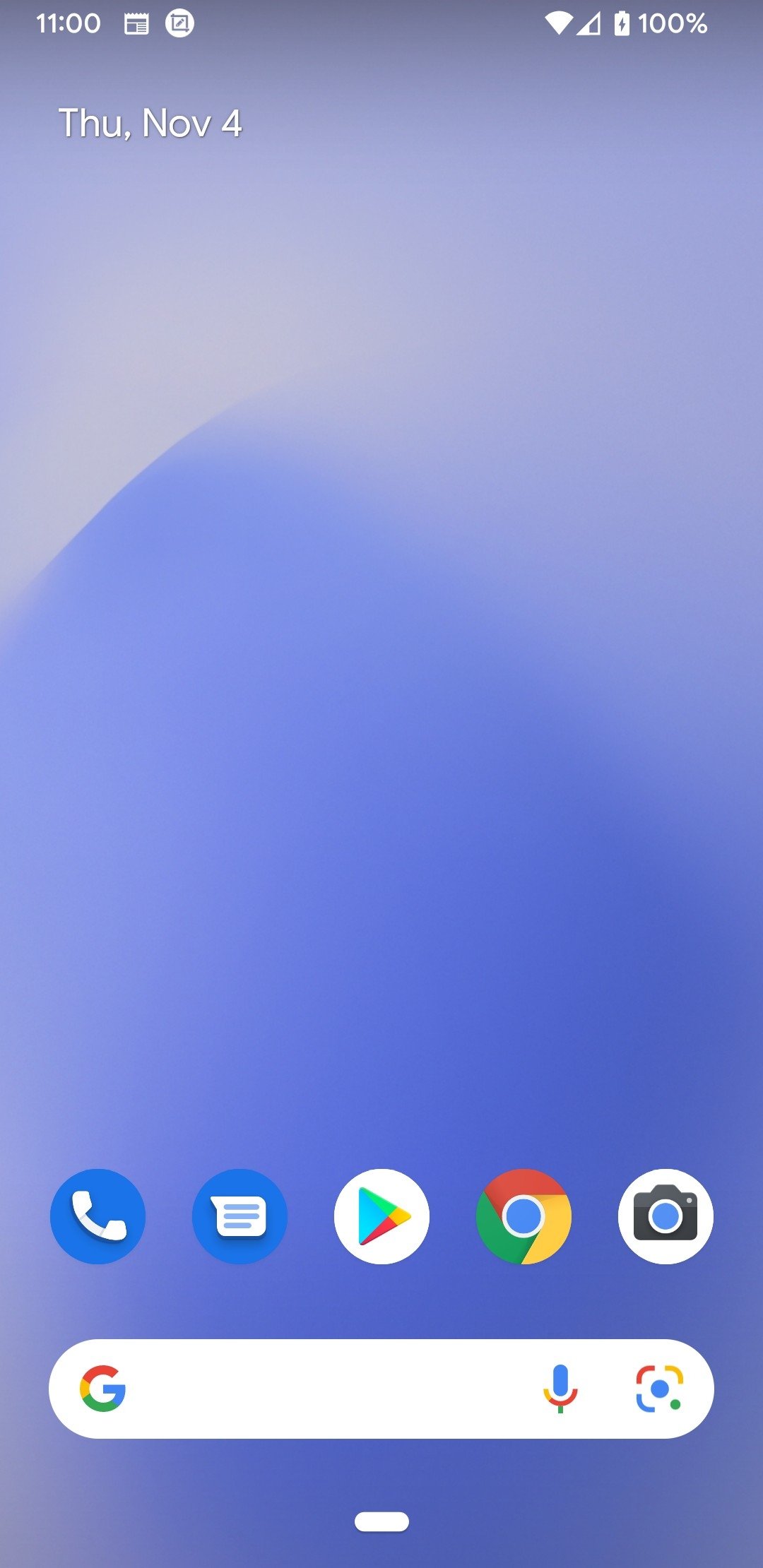This is a cell phone screenshot showcasing the device's home screen with specific focus on elements and icons. The wallpaper is a gradient blend of purple and blue hues, lending a soothing and modern aesthetic to the display. 

On the upper left-hand side of the screen, the time is shown as 11:00. Adjacent to the time is an icon resembling a calendar or a calculator. Next to it is another distinctive icon: a white circle containing a pencil inside a gray box. On the upper right-hand side, typical status icons are present, including the Wi-Fi signal strength icon, the cell reception bars, and the fully charged battery icon at 100%.

Directly beneath the time, the date is displayed as "THU_NOV4," indicating it is a Thursday in November. At the bottom of the screen, a row of essential app icons is neatly arranged. These include the phone's dialer icon, the messaging app icon, the Google Chrome browser icon, the Google Play Store icon, and an icon linked to the photo or gallery app.

The central area of the screen is mainly blank, apart from the presence of a Google search bar situated just above the row of app icons, providing quick access to search functionalities.